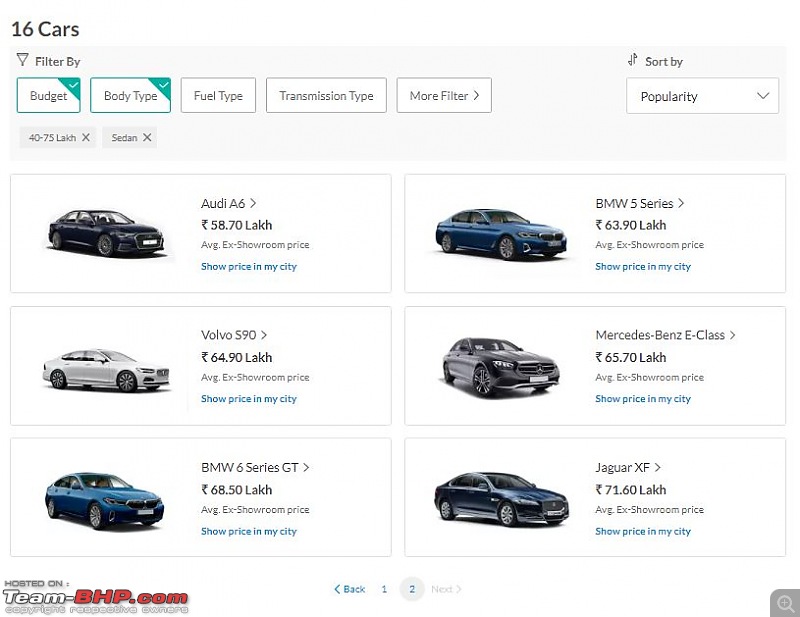This screenshot appears to be from an automobile dealer or sales agent website. In the top left corner, the text "16 cars" is displayed in black font, and just below it, there is a gray horizontal bar. Below this, there is a "Filter By" icon and five rectangular filter buttons: "Budget" with a green triangle in the top right corner, "Body Type" with a green triangle to the right, and "Fuel Type," "Transmission Type," and "More Filters" all in black text on a white background.

On the right-hand side, there is a "Sort By" section with the word "Popularity" inside a white box that features a gray drop-down arrow on the right.

The main section of the screenshot displays two columns with three rows of car listings. Each row features a car image on the left with the car’s name and description to the right. In the top row, the left car is an Audi A6, and the right car is a BMW 5 Series. The second row features a Volvo 590 on the left and a Mercedes-Benz E-Class on the right. In the bottom row, the left car is a BMW 6 Series GT, and the right car is a Jaguar XF. All prices appear to be listed in a currency labeled "LAKH."

At the bottom left of the image, the website is branded with the text "Hosted on" followed by the word "TEAM" in large white letters outlined in black, "DASH" in the same style, and "bhp.com" in red letters also outlined in black. Centered at the bottom of the image are pagination controls: a blue back arrow, the blue word "back," a blue number "1," a blue number "2" inside a gray circle, and a muted gray "next" with a right arrow.